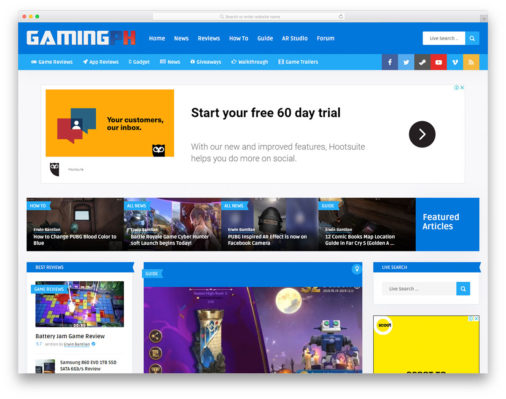This screenshot, taken on a MacBook, showcases the distinct red, yellow, and green buttons on the upper left-hand corner indicative of Apple's interface. Dominating the center is a search bar flanked by the GamingPH logo, which is in white text with a blue "P" and red "H". The top section is divided into two blue segments, with the upper one being a darker shade. This area hosts navigation links including Home, News, Reviews, How-To, Guide, AR Studio, and Forum.

Directly beneath this, there is a secondary search bar enabling live search functionality. The following section in a lighter blue shade features seven unreadable options. Social media icons for Facebook, Twitter, YouTube, Venmo, and a couple of unidentified platforms are also present.

A prominent advertisement occupies the left-center position of the screen. It is encapsulated in yellow with the message, "Your customers are in box. Start your free 60-day trial with our new and improved features. Hootsuite helps you do more on social." A black clickable button with a right-pointing arrow accompanies this ad.

Below, the interface displays four featured articles, each accompanied by a photo. Despite the text being blurry, these articles are visually emphasized. Further down is another article, presumably titled "Game Rewards," featuring an image depicting a moon and a robot.

To the right of this section is another live search tool, including a fill-in area for user queries. The bottom right corner showcases an additional yellow-hued advertisement for Scout.